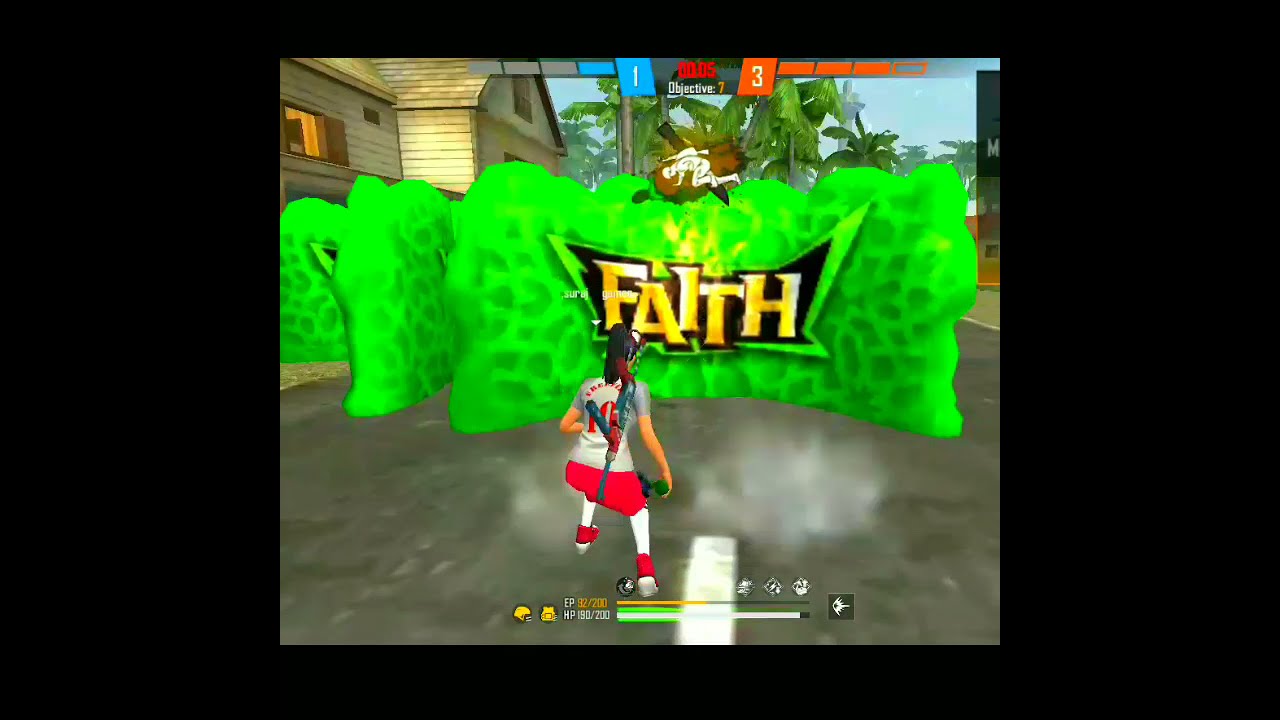The image is a detailed screenshot from a video game framed by a black rectangle, making the actual game screenshot smaller and centered within. A significant element is the presence of three green cloud-like formations arranged with one directly in front, another at an angle behind it, and a third further back. The primary green cloud features the prominently displayed word "FAITH" in yellow capital letters with a black outline. 

In the foreground, a girl stands with her back to the viewer. She is wearing a white and gray sporting shirt, red shorts, and red shoes with white socks. Her long brown hair is visible under a baseball cap, and she appears to have a gun strapped to her back while holding a green canister in her right hand. She stands by a white line painted on the floor. Surrounding her, at the bottom of the image, is a ticker displaying some numbers and progress bars.

At the top of the screenshot, the word "OBJECTIVE" is shown in white lettering, flanked by a blue square containing the number "1" and a red square with the number "3". Additional details include sections of a street with a white dotted line, a brown two-story house with windows, palm trees beside it, and an image of a person possibly injured with a knife through them.

The environment suggests a dynamic scene, with the girl ready for action amidst the green explosions and urban backdrop.